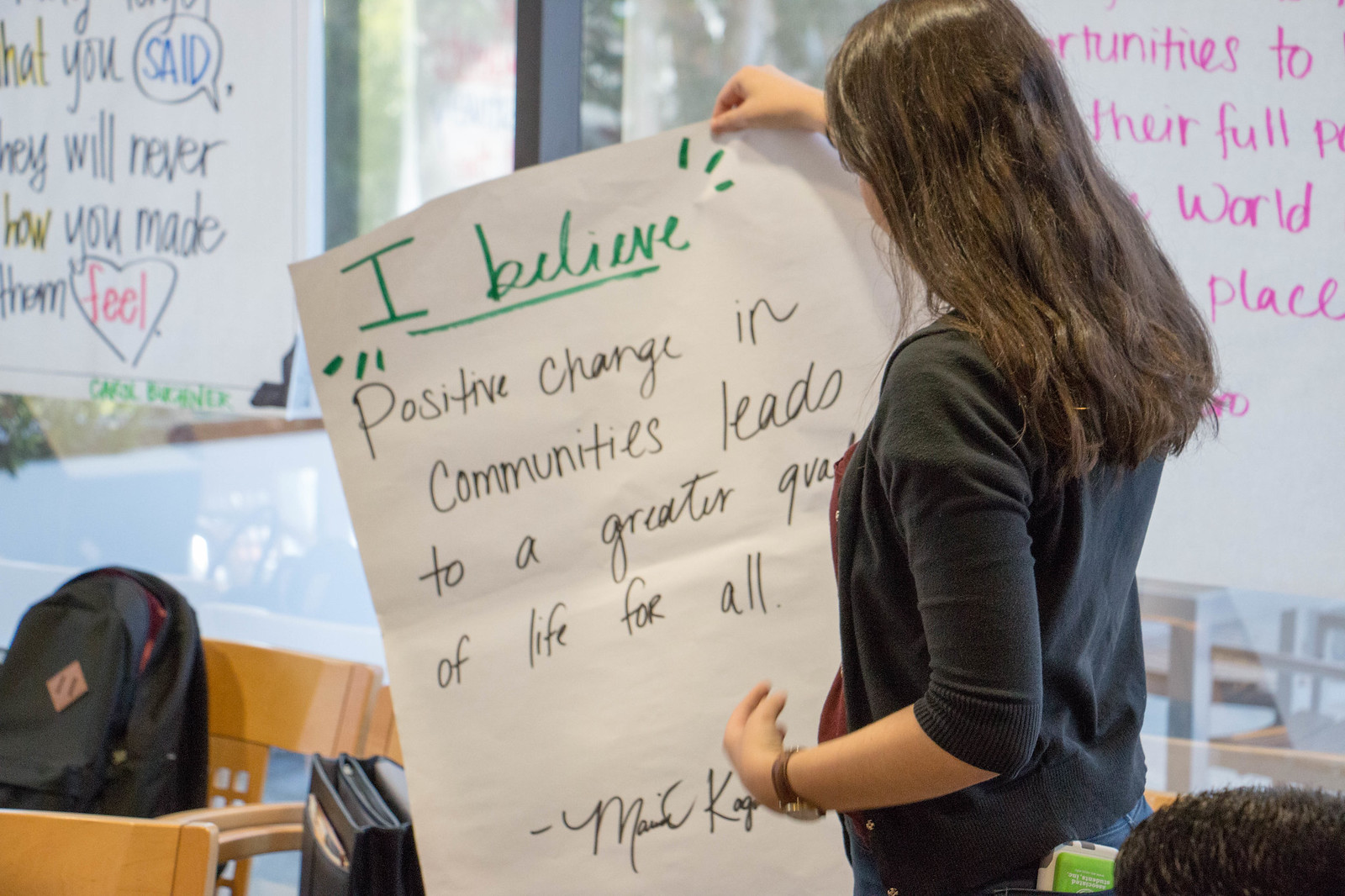In this image, a young woman with long dark hair, dressed in a black or dark navy sweatshirt and sporting a brown wristwatch, stands with her back slightly turned to the left. She holds up a large white piece of paper with green text at the top that reads "I believe," followed by black cursive handwriting that states, "Positive change in communities leads to a greater quality of life for all," ending with a signature that seems to begin with "M" and has a last name starting with "K."

The setting appears to be a classroom or library, characterized by large glass windows lining the far side. Along these windows are various inspirational messages written by students on large pieces of paper and posted up. The space is furnished with light wooden chairs and desks. To the left of the woman, there is a black backpack with a brown diamond emblem on one of the chairs. Additionally, a green object peeks out of her back pocket, and there is a fuzzy dark item behind her. Another bag, which appears brown or black, sits open behind the paper she is holding. Overall, the scene is a collaborative and inspirational environment with students contributing positive messages.